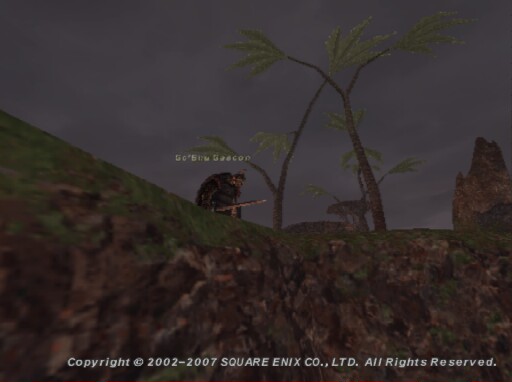The rectangular screenshot, oriented with its long side running from left to right, showcases a scene from a video game. Central to the image is a solitary figure crouched on a hillside, with an unreadable name displayed above. At the bottom of the image, in white text, it reads, "Copyright 2002-2007 Square Enix Company Ltd. All rights reserved."

The backdrop features a dark, tumultuous sky filled with heavy clouds, setting a dramatic tone. The hillside on which the character crouches slopes downward from a higher elevation on the left towards a more leveled area in the middle. The upper portion of the hill is lush and green, while the lower section transitions to rocky terrain. 

The figure, dressed in brown attire, appears to be holding either a sword or a spear. Two trees rise directly in front of the character, partly obscuring the view. In the distance, on the right-hand side, a higher mountain looms, adding depth to the landscape. The overall scene conveys a sense of tension and anticipation against a rugged, natural setting.